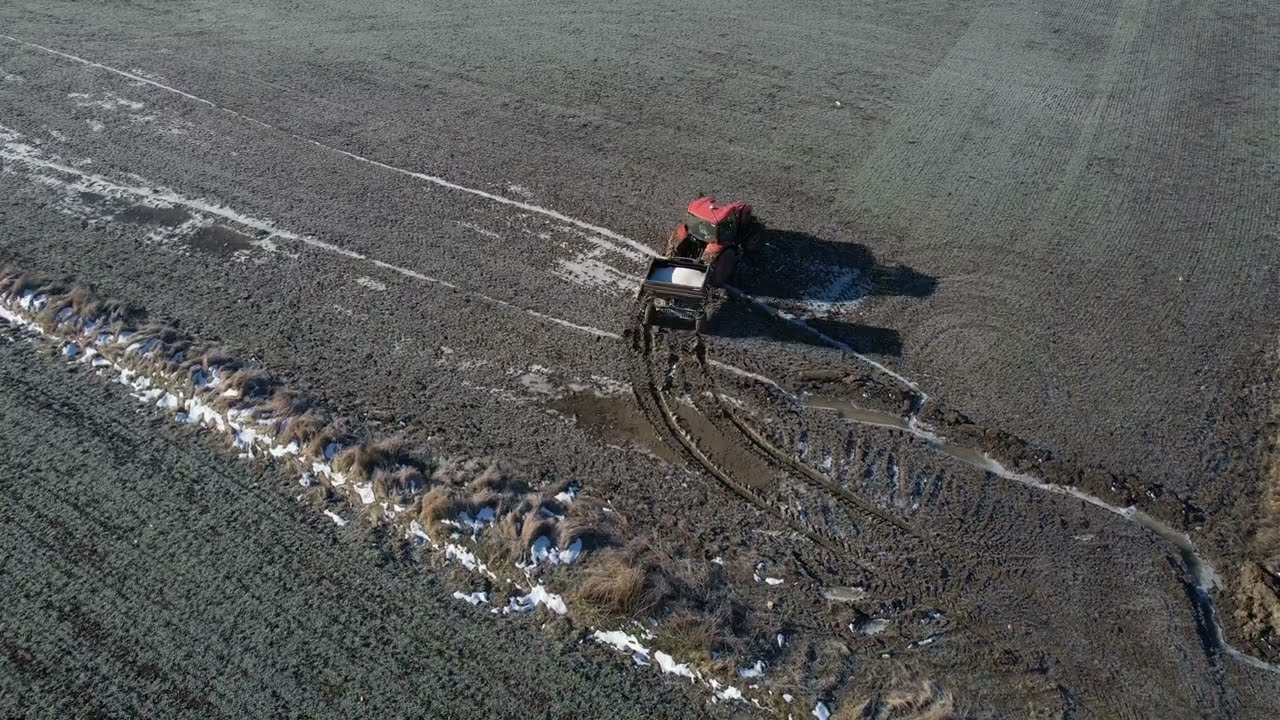The aerial image captures a predominantly muddy and sparsely vegetated field, likely taken during late winter as indicated by patches of lingering white snow. Central to the photo is a red tractor, which appears to be either stuck in or navigating through the mud, pulling a metallic trailer containing a white substance, possibly fertilizer. The trailer leaves distinct track marks and circular patterns in the brown dirt, suggesting the tractor's path through the field. The landscape is predominantly brown and black, indicative of wet, soot-colored mud, with sparse greenish tinges of grass. The photo also captures a contrast between the muddied area and a mossy, darker green field in the bottom right corner, separated by small brown bushes. The lack of visible sky and overall composition suggests the image was taken during the day, focusing downward from above.